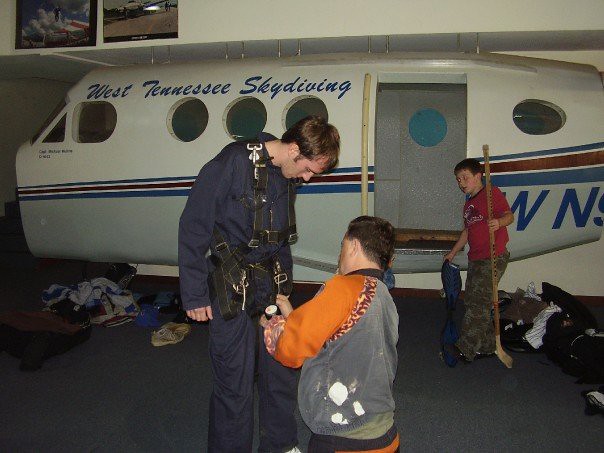This color photograph, taken in landscape orientation, captures the vibrant interior of an aerospace museum or an indoor hangar-type facility focused on skydiving training. Dominating the background is a skydiving plane labeled "West Tennessee Skydiving" in blue script lettering along its top white fuselage. The plane also features red, white, and blue stripes under its porthole windows, some of which appear to be missing their glass. Both the doorway and an additional window of the plane are open, revealing its interior.

In the foreground, two individuals are central to the scene. On the left, a man in a dark blue jumpsuit is being outfitted with a skydiving harness. He looks downward at a crouching man who is adjusting the straps; this man wears an orange-sleeved shirt with a gray body. Both appear intensely focused on securing the skydiving equipment.

In the background near the plane, a boy dressed in a red t-shirt and camo pants carries what looks like a hockey stick and a blue bag. His position at the steps onto the airplane suggests he is not directly involved with the other two individuals. Scattered around him and on the ground to the left side of the plane is what appears to be laundry or perhaps parachutes sprawled out from suitcases.

The overall ambiance of the photograph indicates a busy and detailed preparation for a skydiving activity within a well-equipped training environment. The training fuselage, seemingly suspended by struts from the ceiling, adds to the authenticity of the setting, which is accentuated by a low ceiling with a few posters visible on a white wall in the background.